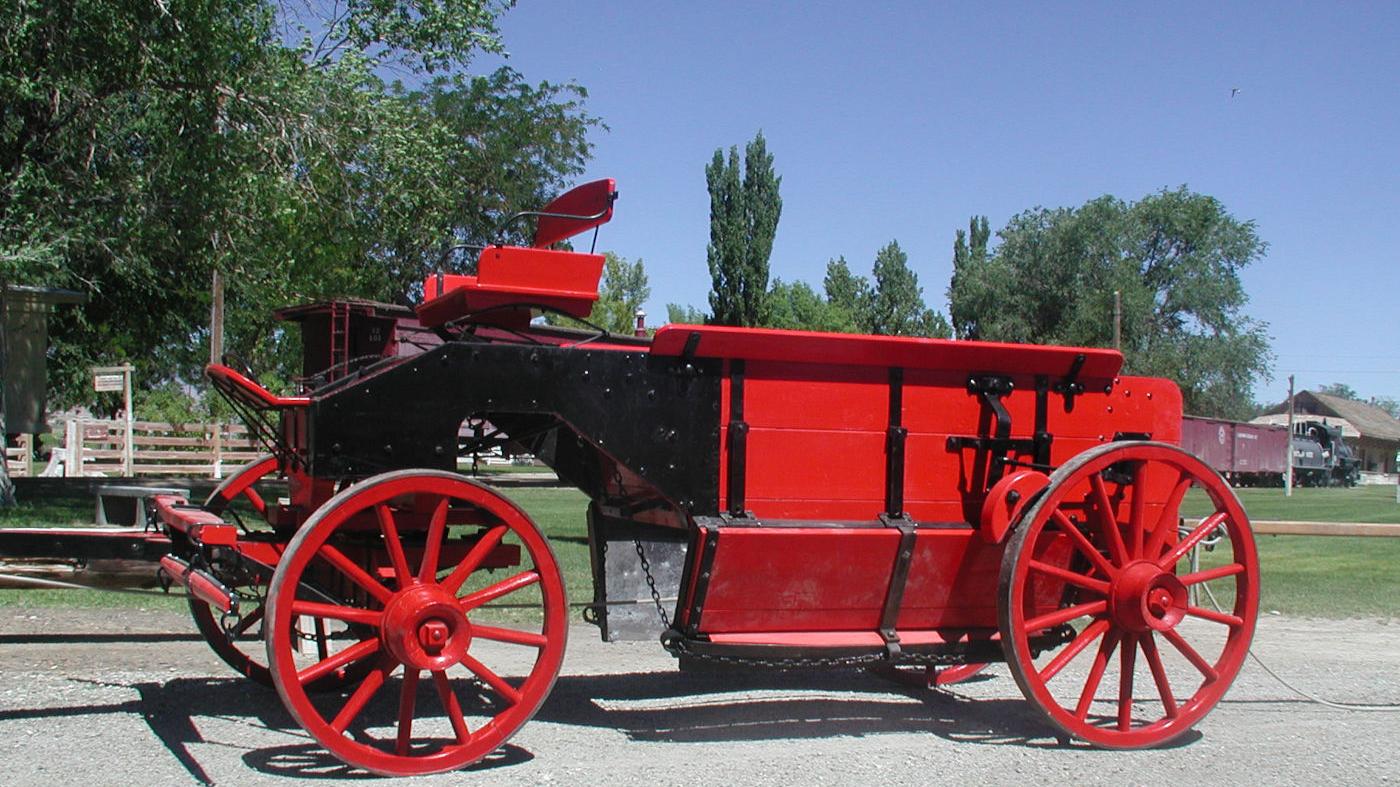In this vibrant landscape image, the focal point is a meticulously painted red and black carriage prominently situated on a stretch of pavement. The carriage, primarily painted in a striking red, features large red wheels with black-edged rims, adding a distinct contrast. The open seat at the front, roomy enough for two, is accented with metal handles, further enhancing its vintage charm. The lower part of the carriage displays black metal sides, providing a subtle yet striking contrast to the vivid red. In the backdrop, a serene setting unfolds with lush green trees and a clear blue sky. There is a patchwork of elements, including a wooden fence to the left, a quaint little building with a red roof, what seems to be train cars or possibly trash containers, and a truck, all hinting at a rustic yet lively ambiance. The pavement extends towards a white fence partially visible amid the greenery, capturing the essence of a peaceful countryside scene. The entire scene is bathed in sunlight, creating shadows that add depth and a touch of realism.